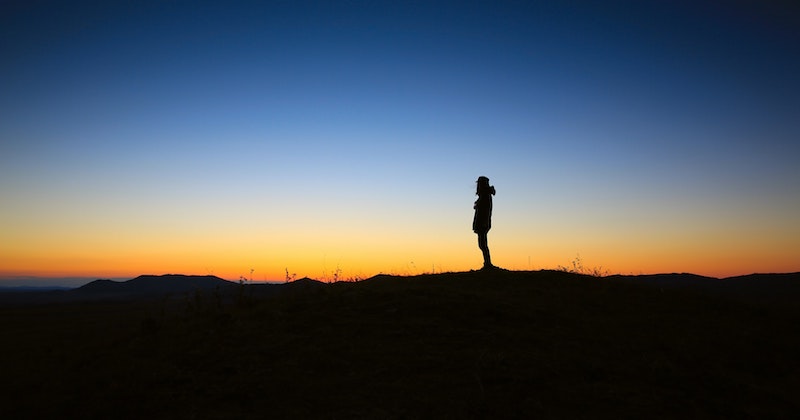This wide-angle photograph captures a tall, thin silhouette of a person standing atop a low hill or ridge, running the entire width of the image. The figure, possibly a hiker outfitted with a jacket, slacks, and a small hat, also appears to have a hood and possibly a backpack or photographic equipment over their shoulder. It is either dawn or dusk, with the sky showcasing a beautiful gradient: the bottom third is black, representing the shadowy land; the middle section transitions into a yellowish-orange band from the just-set or emerging sun; and the top half shifts into a dark blue sky. Silhouettes of vegetation around the ridge add depth to this serene, panoramic view.